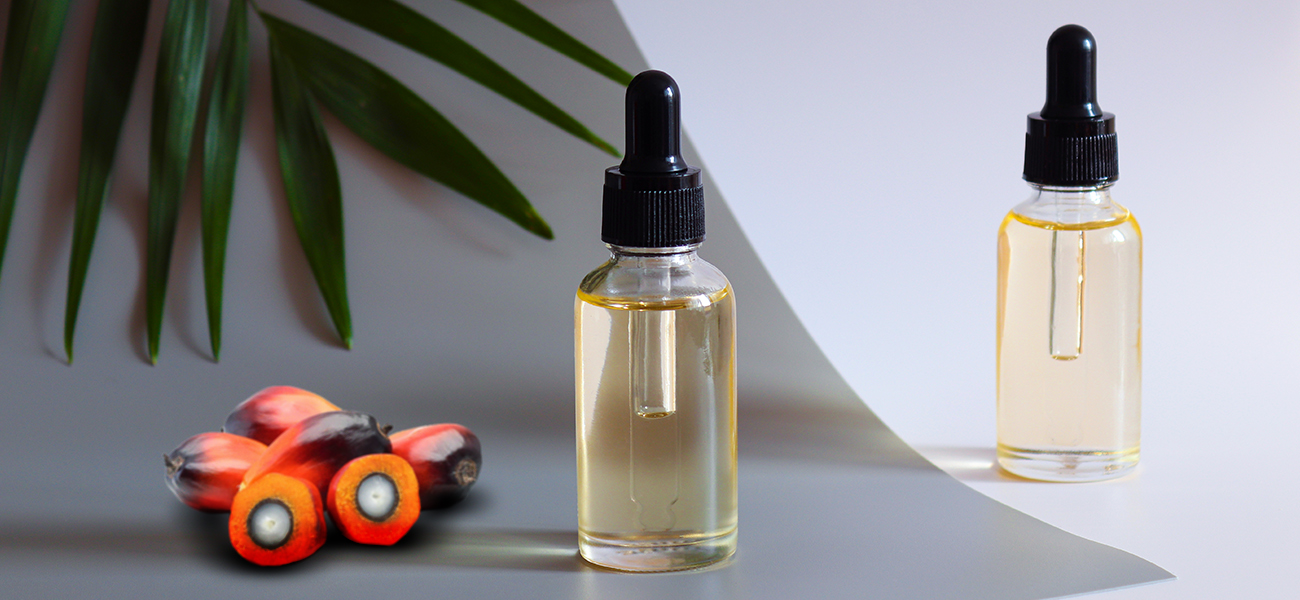The image features two clear cylindrical spray bottles, each topped with a rubber droplet apparatus akin to those found on baby bottles or pacifiers. The droppers are black with a rubber top, allowing for individual liquid drops. Both bottles are filled with a pale, peach-colored, somewhat opaque liquid. They are set in a pristine white environment. Adding a touch of nature to the scene, the top left corner is adorned with several green leaves shaped like small ovals, totaling seven or eight in number. At the bottom left, organic-looking berries, resembling orange and black nuts or possibly toasted acorns, are displayed, some of which are cut open to reveal their white insides. The image is underscored by an all-white background, enhancing the stark contrast and detail of the objects pictured.